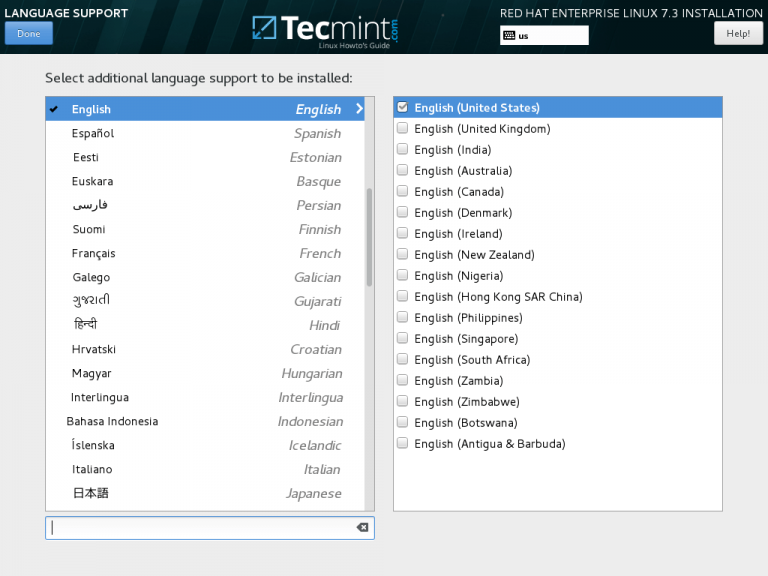This is a screenshot of the language support page on the website TechMint.com. The page features two prominently displayed tables against a light grey background. 

The table on the left lists various languages with English at the top, highlighted and selected. Below English, several languages starting with the letter 'E' are displayed, including Español (Spanish), Eesti (Estonian), Euskara (Basque), and also other languages like Persian, Suomi (Finnish), and Français (French).

The table on the right, a submenu triggered by the selection of English in the left table, lists different variants of the English language specific to various countries. The top selection is English (United States), followed by English (United Kingdom), English (India), English (Australia), English (Canada), English (Denmark), and English (Ireland). This table continues to list approximately 15 different English variants.

Both tables are set within white text boxes that stand out against the light grey background, providing a clear and organized view of the linguistic options available on the website.